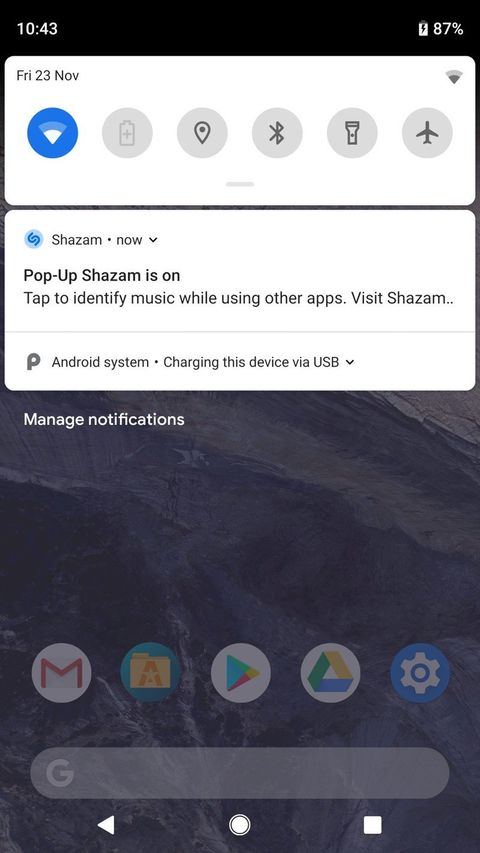A smartphone screen displays a bustling interface, rich with icons and notifications. The user appears to be preparing to use Shazam, an app for identifying music. The Shazam notification is centrally prominent, with a message that reads: "Shazam is on. Tap to identify music while using other apps. Visit Shazam." This notification is nested beneath the bold heading "Android System," which indicates the phone is currently charging via USB. Below, a command prompts the user to "Manage Notifications" in white text.

A series of five app icons are arrayed mid-screen: Gmail, Google Play, a gold folder labeled 'A,' Google Drive, and the phone's Settings. At the bottom of the screen, navigational controls include a search bar and white icons for a browser (←), home (o), and active apps (□).

The top-left corner of the screen shows the time is 10:43, and battery life is at 87%, positioned to the right. An active Wi-Fi icon glows blue, while a set of deactivated icons for Flashlight, Bluetooth, and Location Services remain greyed out. The date is highlighted as Friday, November 23rd.

The visual appeal of the interface is complemented by a scenic wallpaper depicting a majestic rocky mountain with a cascading waterfall, adding a touch of natural beauty to the technical tableau.